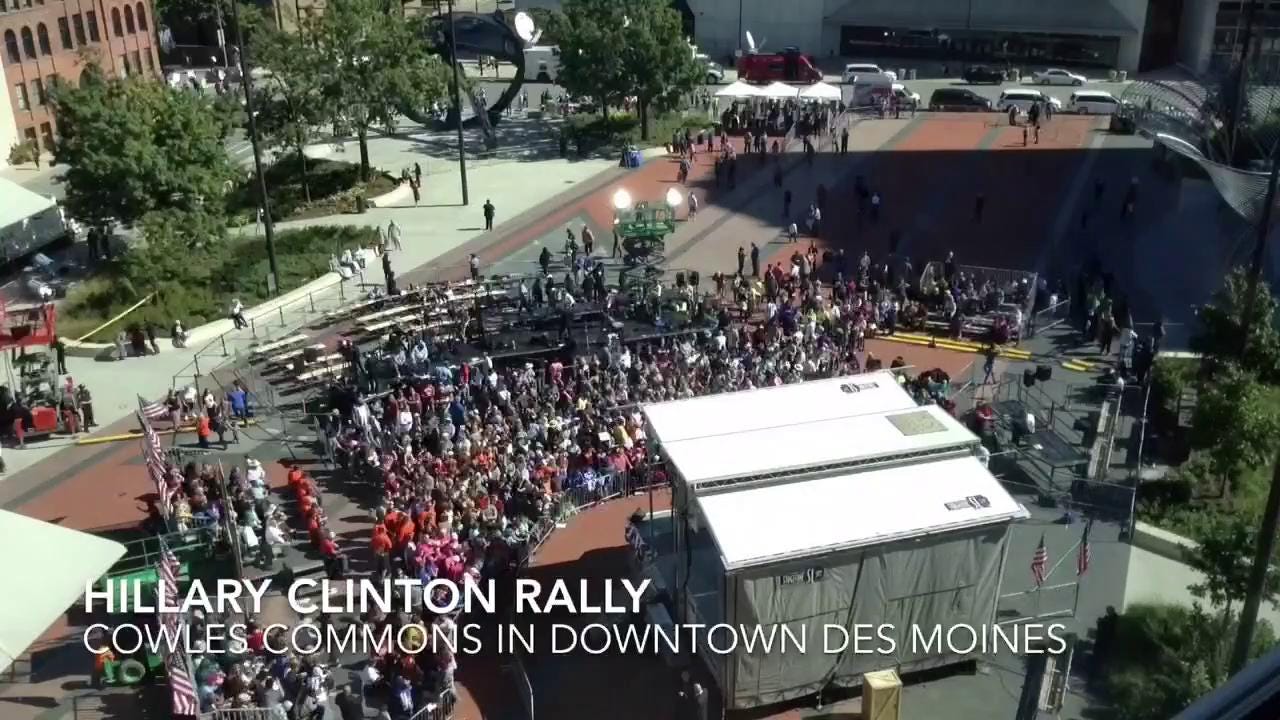This is an overhead view of a Hillary Clinton rally at Cowles Commons in downtown Des Moines. The image captures a sizable crowd of several hundred people gathered in an outdoor setting. The lower left-hand corner of the image bears the text "Hillary Clinton Rally, Cowles Commons, downtown Des Moines." The scene includes bleachers or seating areas where people are either standing or sitting behind barriers. A large, white-topped stage is set up facing the crowd, though only the top of the stage is visible. Surrounding the commons are green areas, visible trees, office buildings, parking lots, and bustling streets with vehicles. Chain link fences are erected to manage crowd flow and keep the area secure. Vendors are present along the streets, and news vans equipped with satellite dishes are parked nearby. Despite some varied perceptions of the crowd size, it is evident that the bleachers and seating sections are occupied with attendees.